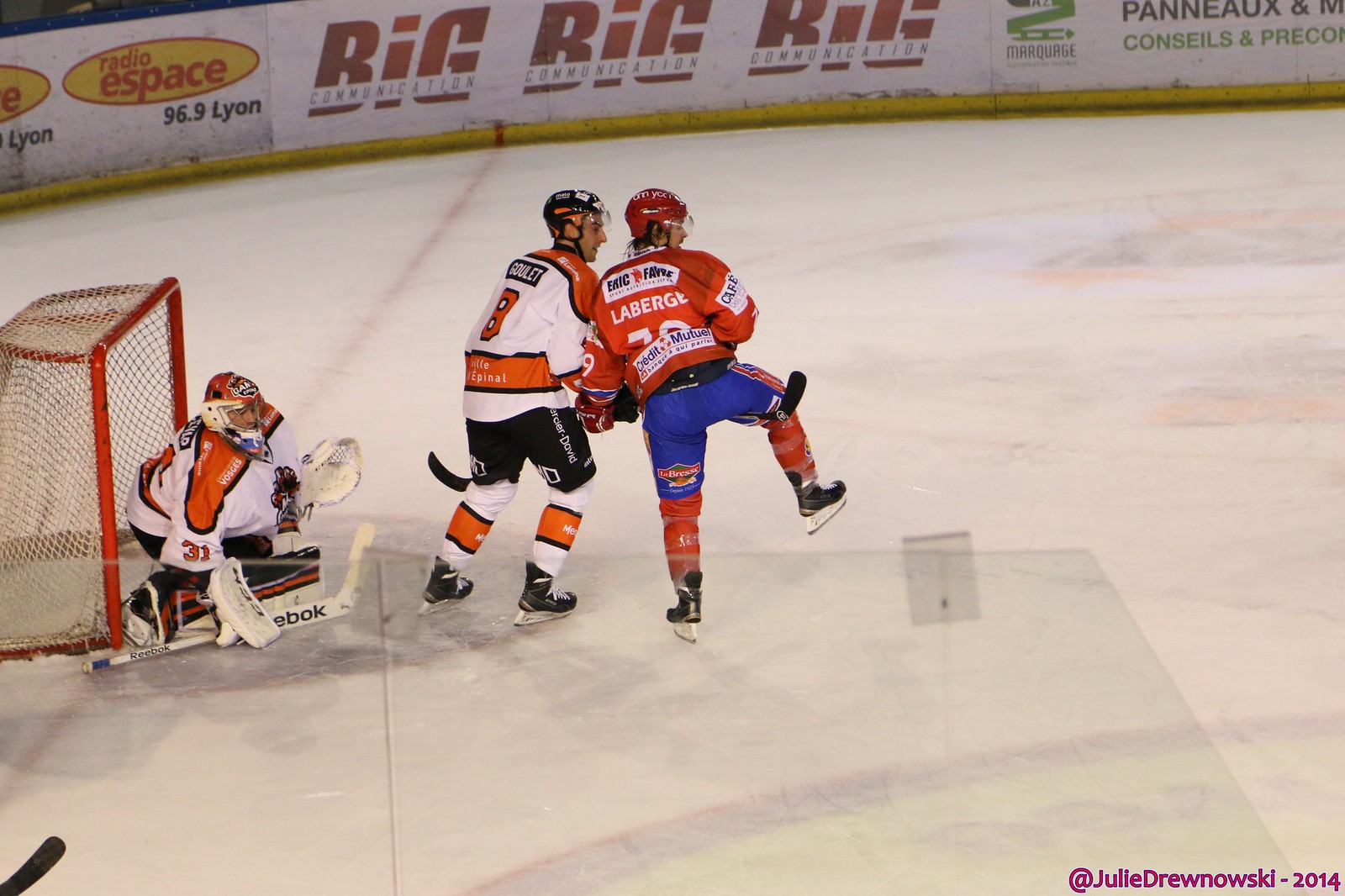This detailed image captures an intense moment during a competitive hockey game at an indoor rink. Dominating the scene are three hockey players, including a goalie positioned to the left and behind a net. The central players, wearing distinct team jerseys, are engaged in a fierce battle: one in an orange, white, and black jersey with black pants and helmet, and the other in red and blue with a red helmet and blue pants. The player in red has his leg raised, entangled with the stick of the orange-clad player. The goalie in the background also sports orange, white, and black gear, including an orange helmet. 

Above the players, the boards are adorned with colorful advertisements in red, yellow, and green against a white backdrop. Prominent text includes "Big Communication," "Radio eSpace 96.9 Lyon," and a partially legible French phrase featuring "Panneaux" and "Conseils." The icy surface of the rink covers the majority of the lower section of the image, with the upper eighth showcasing the ad-covered boards. The scene is framed by the chilly white ice, emphasizing the vibrant and dynamic colors of the players' uniforms. Also noted at the bottom right corner is the copyright "Julie Dronowsky 2014," marking the photographer's credit.